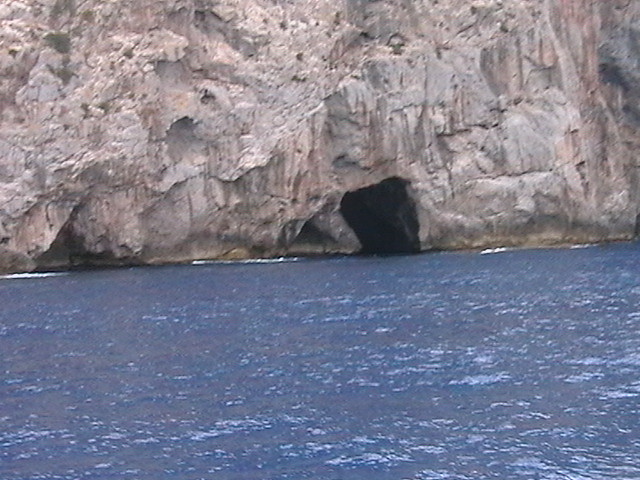In this photograph, you're looking across a body of water that transitions from light to dark blue-gray, dotted with white caps and small waves. The water, though somewhat wavy, is contrasted by the imposing, almost sheer rock wall that dominates the scene. This cliff, with its ledges and pockmarked surface, appears to have suffered from extensive erosion over time, leading to drips and surface irregularities. These erosion patterns have created holes across the cliff face, some of which seem like scars of natural wear. Directly at the base of this formidable rock wall, slightly right of center, lies a mysterious black cave, its entrance swallowing the water but revealing nothing within its depths. The overall image captures the raw and rugged beauty of nature's slow, relentless sculpting.